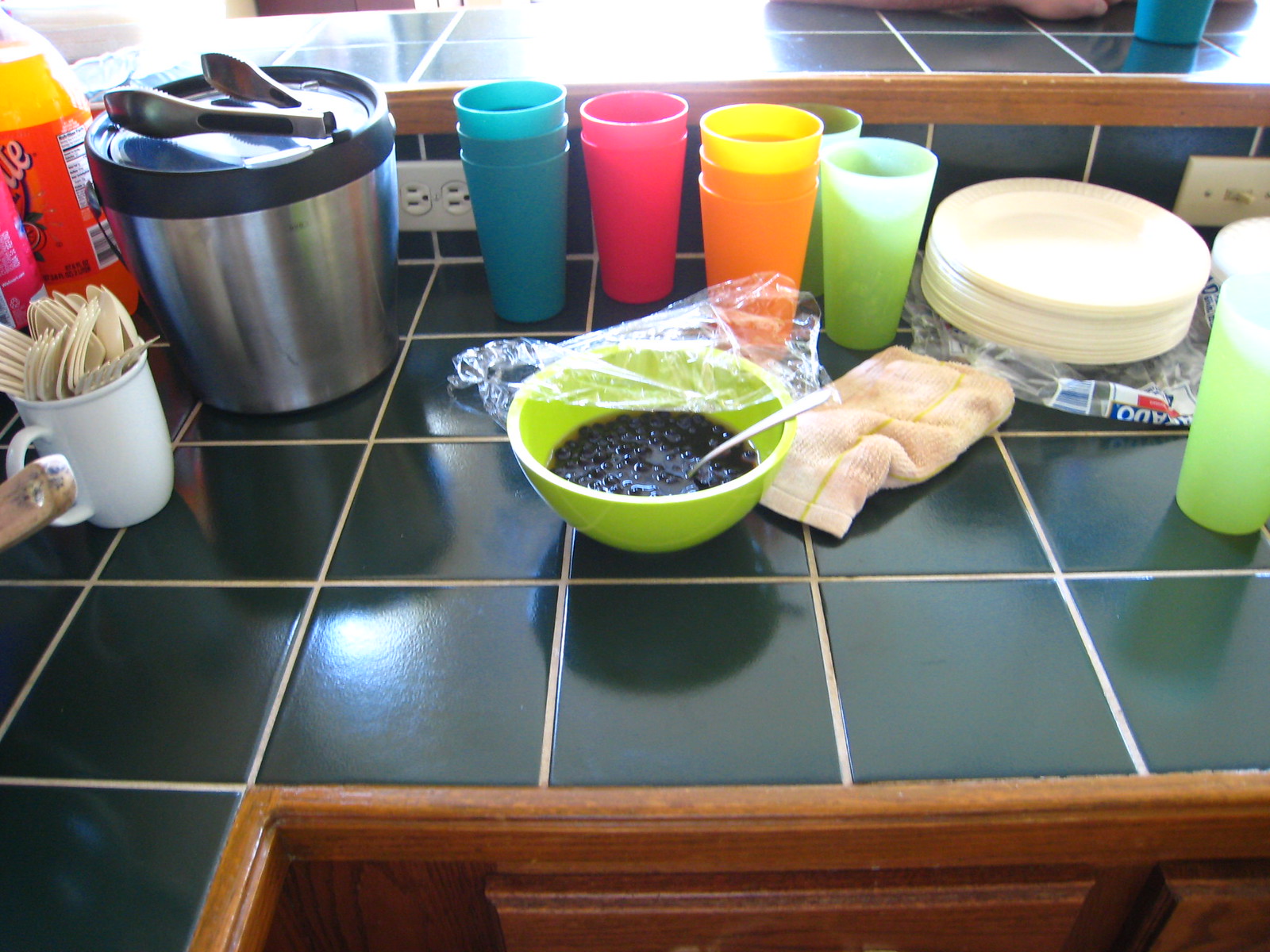The photograph features a kitchen counter with a two-tiered surface, showcasing an intricate design with dark evergreen square tiles. Prominently positioned in the center of the lower level is a lime green bowl containing a black gelatin-like substance, partially covered with cling wrap that is pulled back to reveal a spoon inside. To the left of the bowl, an ice bucket is placed next to a stack of three blue plastic cups. Adjacent to these, there are two pink plastic cups, followed by two orange cups, and a single green cup at the end of the lineup. A coffee mug filled with disposable forks and spoons sits close by, next to a stack of paper plates. The upper level of the counter is framed with a wood trim, adding a touch of rustic charm to the setting.